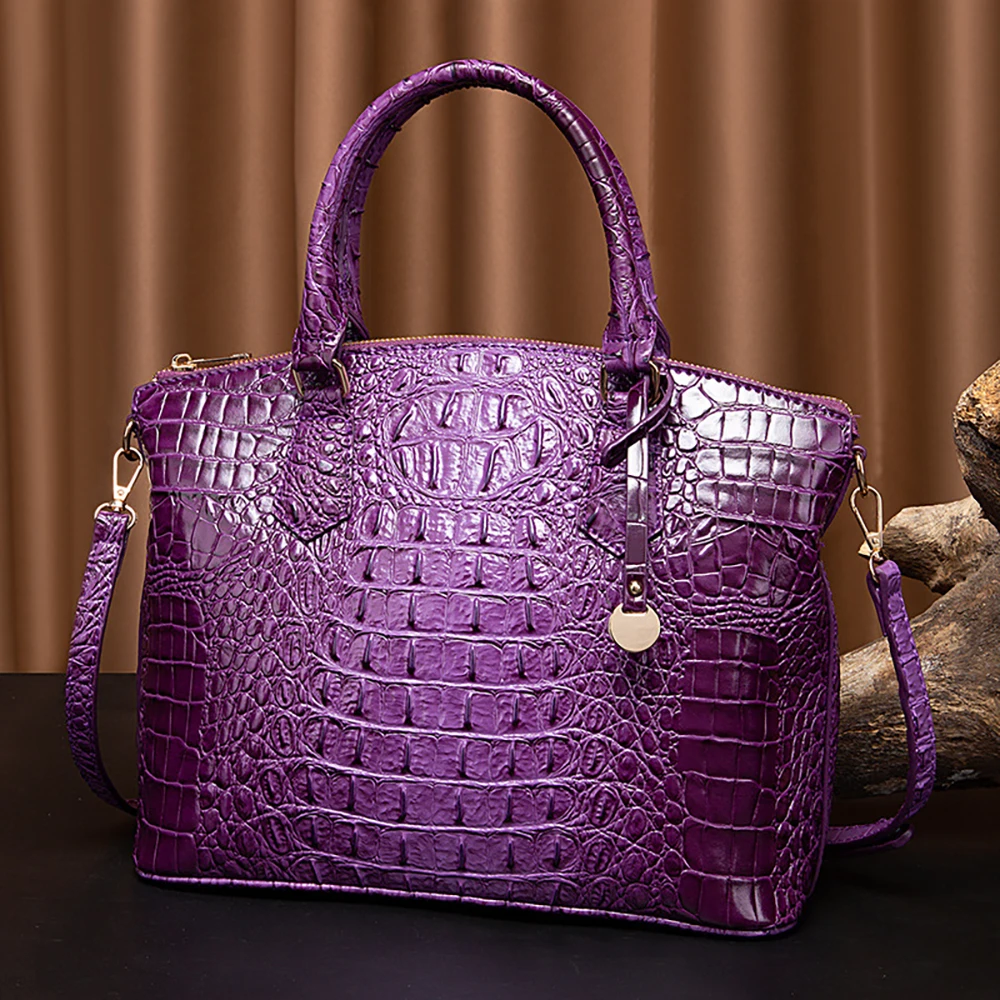The image captures a stylish purple handbag with a distinctive snakeskin or alligator-skin texture. The handbag features a structured design with two short, hard-formed handles and an additional shoulder strap that hangs partially obscured behind the purse. A notable detail is a circular metal dangle attached to one of the handles. The purse is centrally placed on a nearly black surface. The background reveals a brownish-gold, satin-like curtain with varying shades due to its folds, providing a rich backdrop. On the right side of the image, there is a partially visible object, possibly an ornate statue or rock formation, with hues of gold, tan, and brown.